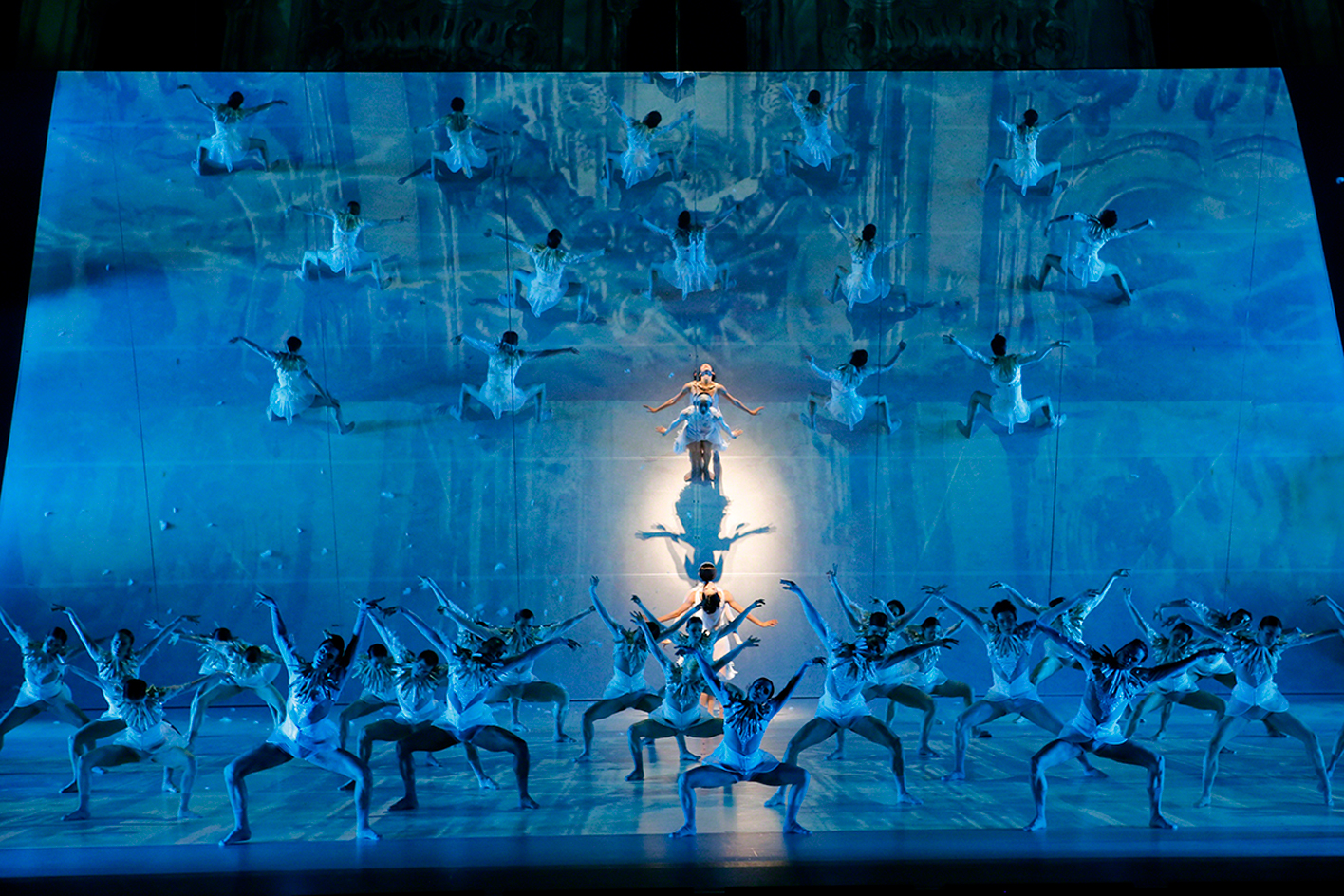The image captures a dynamic scene from a dance production, set against a predominantly blue background that envelops the entire rectangular frame. Around 40 dancers, resembling ballerinas in leotards and ballet shoes, are impeccably synchronized in a pose where they squat on the floor with both arms raised. They are meticulously arranged in rows across the stage, their movements orchestrated to create a cohesive visual spectacle. A large wall, appearing to be a mirror, reflects the backs of the dancers, adding depth to the composition. Amidst this coordinated ensemble, a spotlight singles out a female performer positioned centrally at the back, dressed distinctively in a white gown. This lighting effect creates a striking focal point, highlighting her as the star of the performance. The remarkable stage lighting and blue hues lend the image a surreal, almost cartoon-like quality, making the entire scene visually arresting and meticulously detailed.